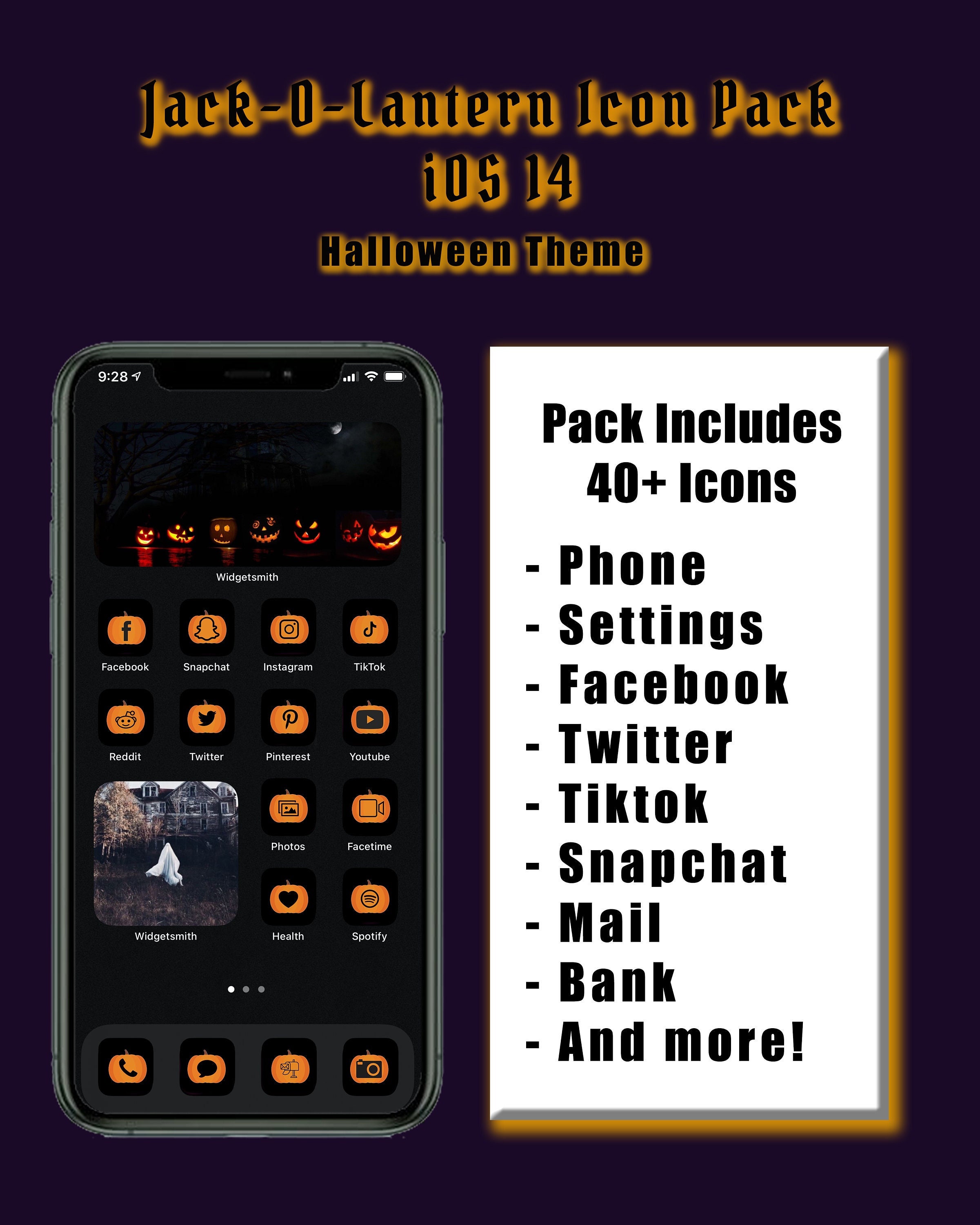A smartphone screen showcases a Halloween-themed icon pack for iOS 14 against a predominantly purple background. The screen is decorated with a variety of jack-o'-lantern icons representing popular apps such as Facebook, Snapchat, Instagram, TikTok, Reddit, Twitter, Pinterest, and YouTube, all depicted as smiling pumpkins. The top-left corner displays the time (9:28) and location services icon, while the top-right corner shows full WiFi and battery indicators. The dark ambiance includes trees and a crescent moon at the top, and numerous pumpkins scattered on the ground, like pickles, numbered 1 through 8. Additionally, a widget reveals a gusty scene with a wooden building and dead grass. The phone status bar shows photos, FaceTime, health, and Spotify apps. A speech bubble and camera icons are visible beside the pumpkins. On the right side, a description touts the pack's inclusion of over 40 icons covering phone, settings, Facebook, Twitter, TikTok, Snapchat, mail, banking, and more. The phone has grey edges with an orange shadow, complementing the overall purple background.